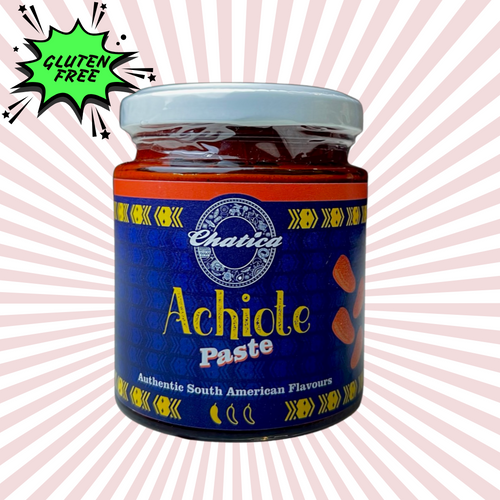This is a detailed close-up photograph of a jar of Achiolete paste branded as Chatitas. The jar has a white screw-top lid and is wrapped in safety plastic. The label features a vibrant design with red, blue, and yellow elements. At the center of the label is a prominent yellow circle with the brand name “Chatitas” in caps for the 'C' and lowercase for the remaining letters. Below the brand name, in yellow letters, it reads “The Anchovy Paste,” followed by the phrase “Authentic South American Flavors” at the bottom. The background of the image is a white canvas with light pinkish rays extending to each corner, giving a starburst effect. A green burst in the upper left corner contains the words "Gluten-Free" in black text. On the label, there is a yellow stripe and illustrations of three small red peppers at the bottom, hinting at the spicy red paste inside the glass jar.